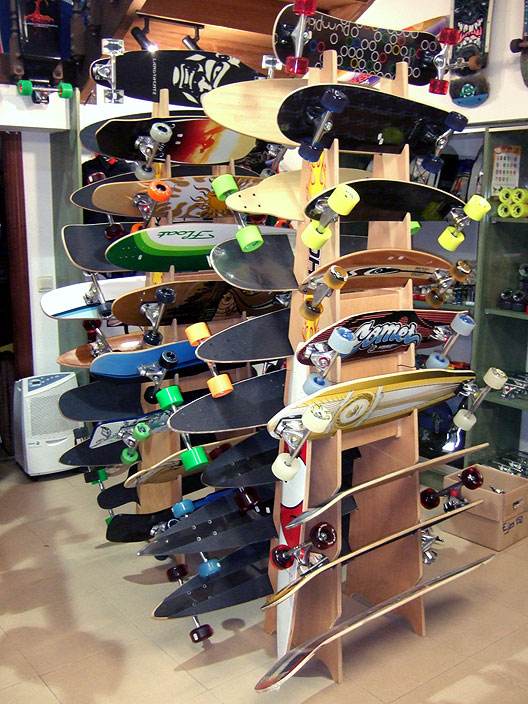In the image, we see the vibrant interior of a skateboard shop with a beige-tiled floor. Dominating the center are two large wooden stands, each holding a total of 18 skateboards - nine on the front and nine on the back - set at an angle. The boards themselves mostly have black tops and feature a dazzling array of colorful designs on the undersides, accompanied by wheels in neon green, neon orange, white, yellow, and red, making for a lively display.

To the right of these central stands, there is a display case showcasing various skateboard wheels and accessories. The stands themselves appear to be wooden and brown, perfectly matching the shop's rich, wooden aesthetic. In the background, we also notice additional skateboards mounted high up on the wall, adding to the shop's vibrant, bustling atmosphere.

The left side of the image reveals a humidifier on the floor, along with a brown door partially visible. This detailed setup situates the viewer inside a well-stocked, colorful retail space bustling with skateboard variety and accessories, set against the backdrop of a shop with a distinctive brown and beige color scheme.